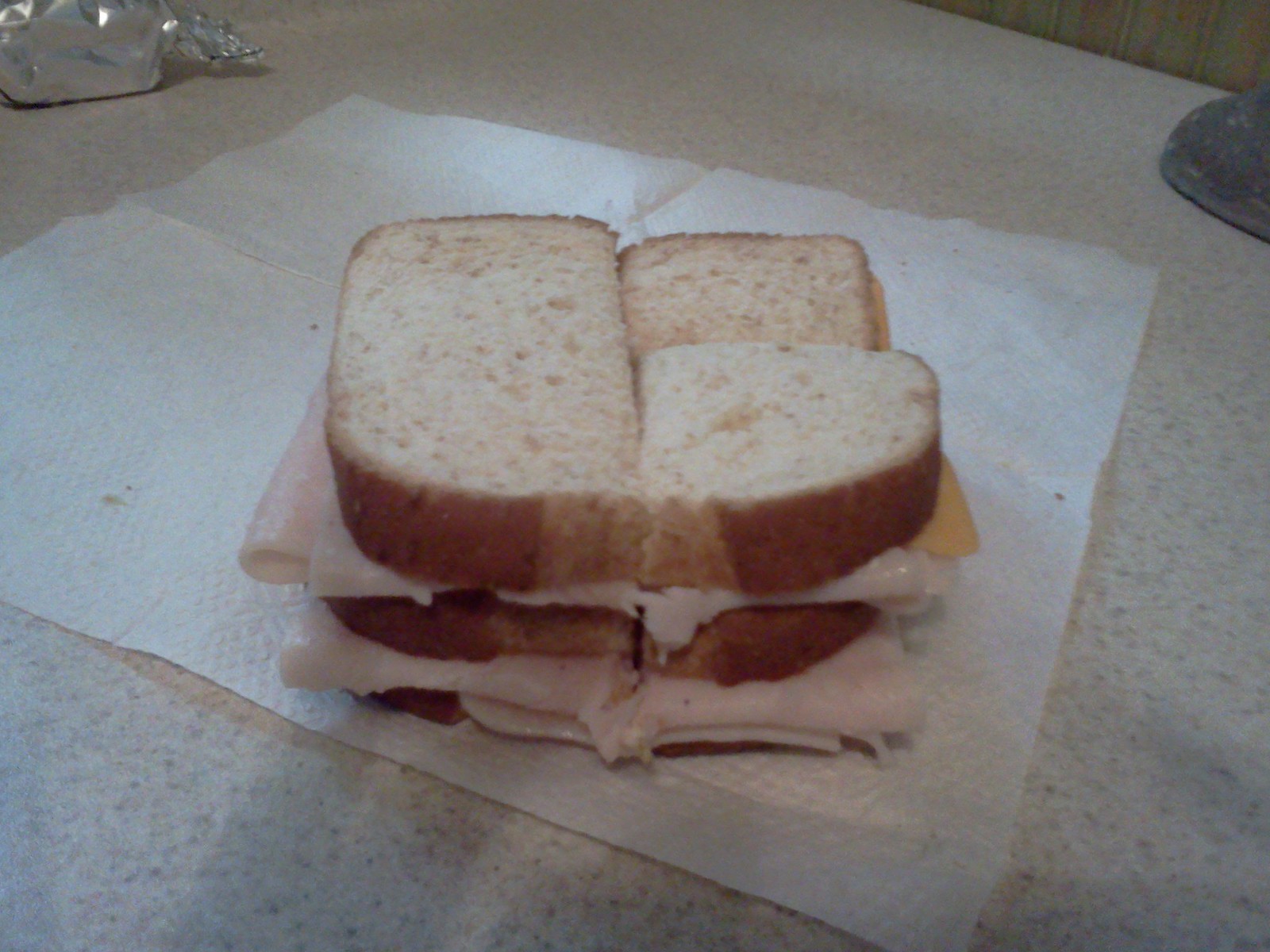The photograph captures a detailed view of a lunch setting, focusing on a sandwich placed on a white, unfolded paper napkin that occupies a considerable portion of a speckled granite-like countertop. The sandwich is made of three slices of plain bread, layered with shredded turkey deli meat and a slice of yellow cheese, and is cut into three pieces—first halved, with one of the halves further divided. In the top left corner of the image, there is a crumpled piece of aluminum foil. The background also reveals a section of wood grain on the wall and what appears to be another foil-wrapped object partially cut off by the edge of the image. Scattered crumbs can be seen on the napkin around the sandwich.